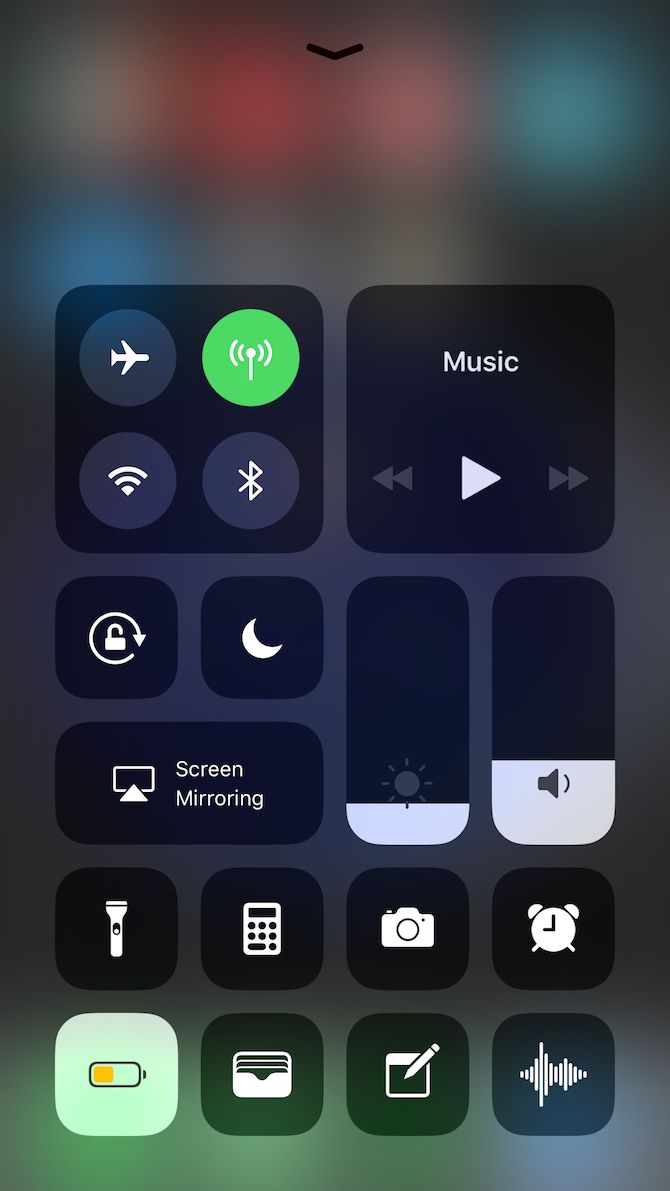This is a screenshot of an iPhone's pull-down control center menu, displayed over a blurry home screen background. The pull-down menu showcases various settings and controls. At the top left, there are four circular icons: Airplane Mode (enabled), Mobile Data (enabled), Wi-Fi (disabled), and Bluetooth (disabled). To the right section, there is a music control panel with play, skip back, and skip forward buttons.

Below the primary options, there's a brightness control bar set to approximately 10% and a sound volume bar set to around 30%. Under these, there are additional icons: a timer symbol, a speaker icon possibly related to music control, a camera icon, and a notes app icon. 

Beneath the top four circles, there are more control icons: Screen Orientation Lock, Do Not Disturb (crescent moon), Screen Mirroring, Flashlight, Calculator, Power Saver Mode (which is enabled), and a File Management button.